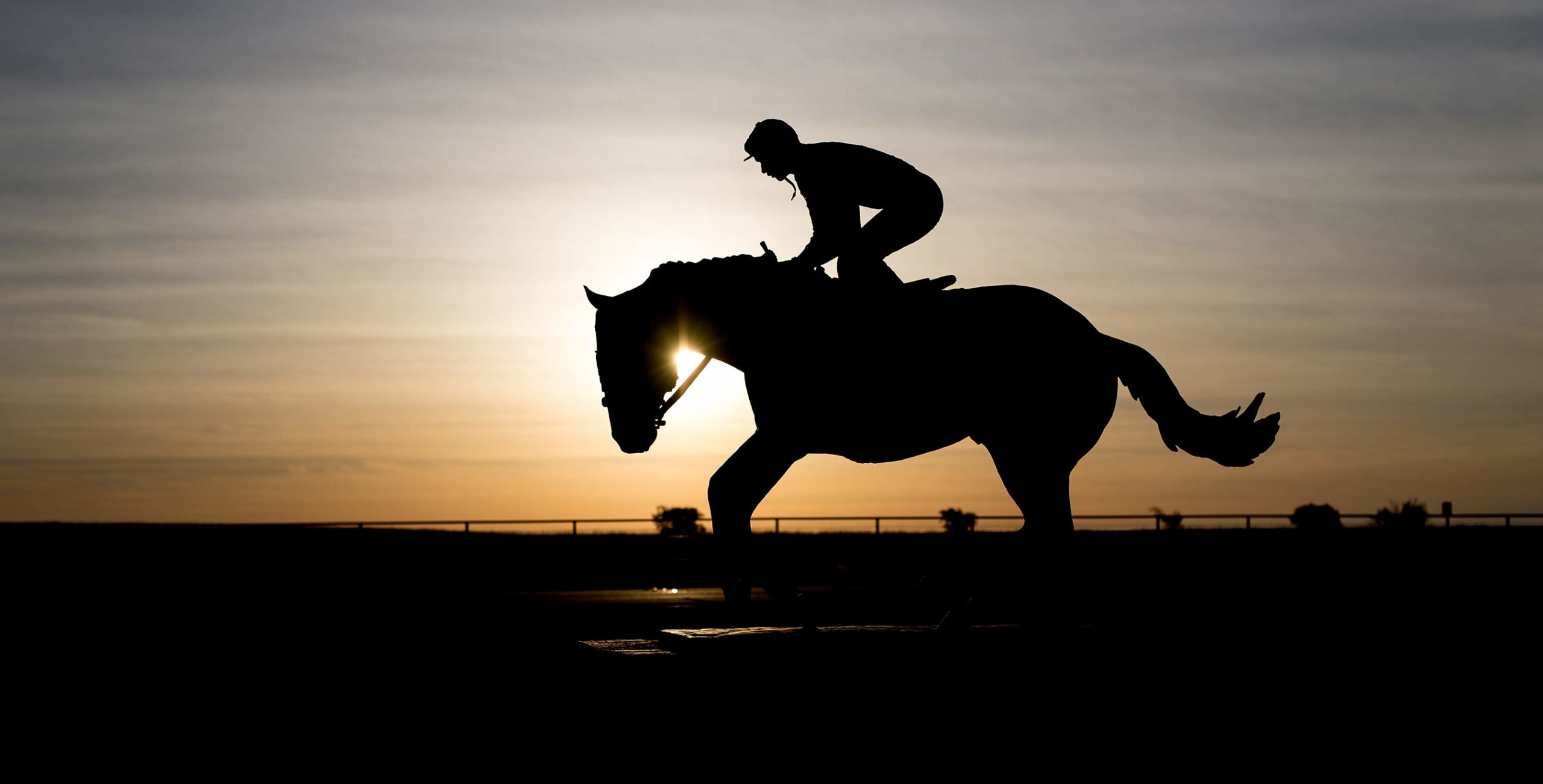The photograph captures the striking silhouette of a jockey riding a racehorse at sunset. The sky, awash in a blend of orange and gray hues, serves as a dramatic backdrop to the scene. The sun peeks through the gap between the horse's neck and jaw, casting a brilliant flare that enhances the golden ambiance of the horizon. Both the jockey and the horse are immaculately silhouetted, with notable details like the jockey's helmet with a dangling chin strap, the tightly pulled reins, and the horse's tail flowing behind as it appears to be in motion. The ground beneath them is entirely black, accentuated only by subtle reflections suggesting the presence of small puddles. A finely trimmed, short-cut grass field and a slender fence with a few scattered bushes further define the setting, possibly indicating a racetrack. The overall composition of the image is both dynamic and serene, capturing the ephemeral beauty of the sunset while highlighting the silhouette of the horse and rider in perfect harmony.